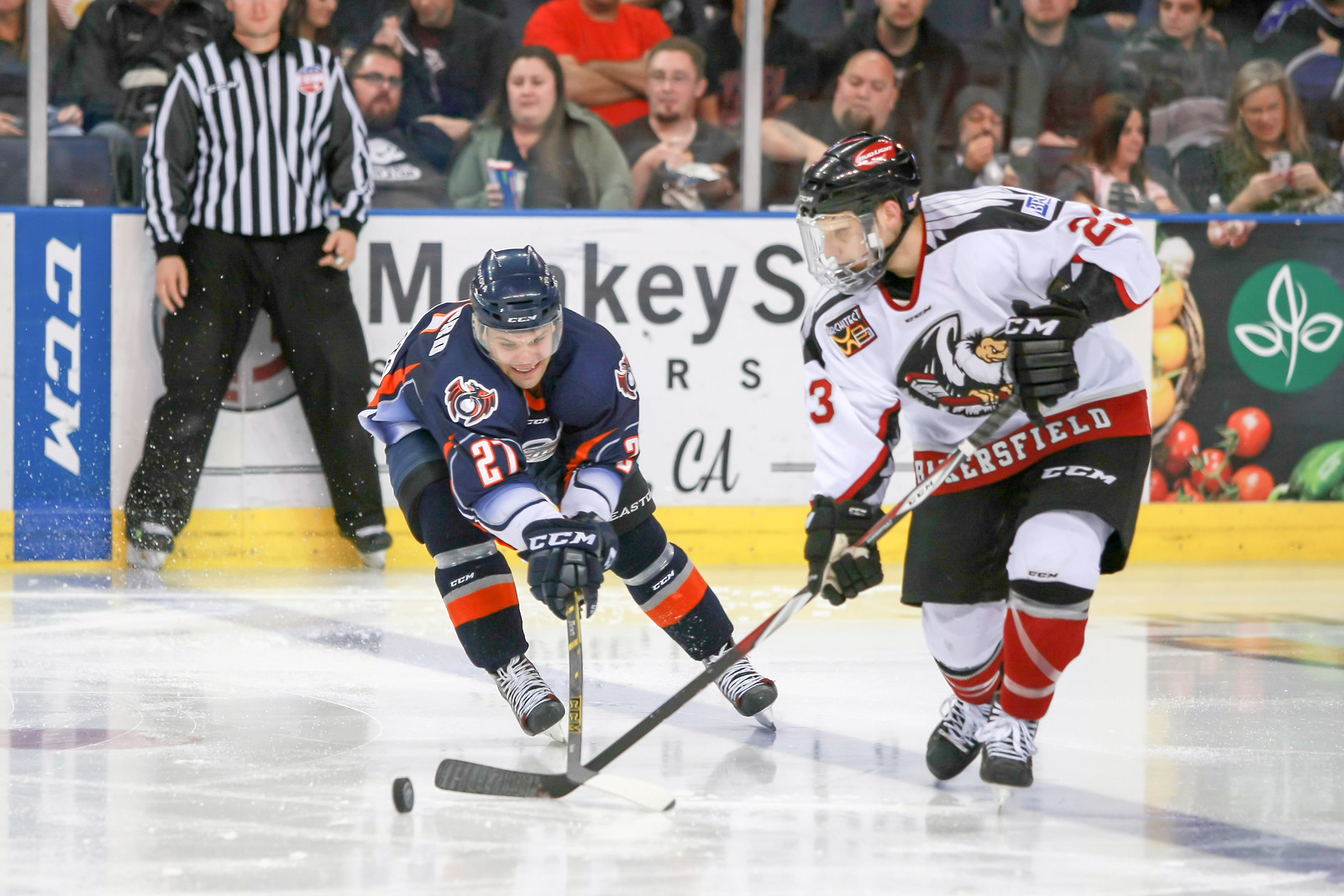In the image, two ice hockey players are intently battling for a puck on the ice. The player on the left is dressed in a navy blue jersey with orange detailing, black pants, and a blue helmet, extending his hockey stick toward the puck. The player on the right wears a white jersey with red and black accents, black shorts, and a black helmet with red details, also focusing on the puck. Both players are fully engaged, their sticks clashing as they fight for control. In the background, a referee stands against a back wall adorned with advertisements; he wears a black and white striped shirt and black pants, with his face partially cut off in the image. The visible part of the advertisement appears to say "monkeys." Behind the referee, a row of fans in the stands watches the game intently, some holding snacks or looking at their phones.